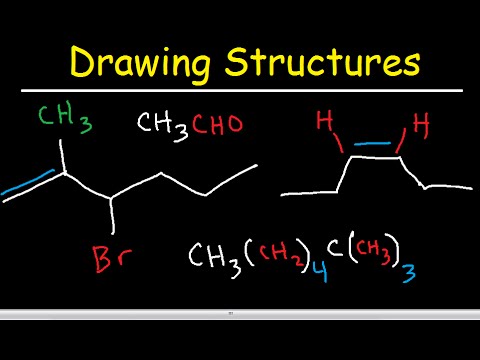The image is a screenshot from an organic chemistry lecture or slideshow, with a black background. At the top, in a bubbly yellow font, the title "Drawing Structures" is prominently displayed, followed by a thin white line. Below this, there are various molecules and chemical formulas depicted, each color-coded. "CHO" is marked in red, "CH3" appears in green, and another "CH3" is in white. Each element, including hydrogen (H) and bromine (Br, in red), is connected by colored lines illustrating chemical bonds, both red and blue. Further down, between a top thin white line and a thicker bottom white line, there are two distinct compounds. The first involves "CH3" and "CH3CHO" connected to "Br". The second complex formula involves "CH3CH2" with additional H atoms and repeats of "CH3". The colors and lines together form a detailed visual of drawing chemical structures in organic chemistry.